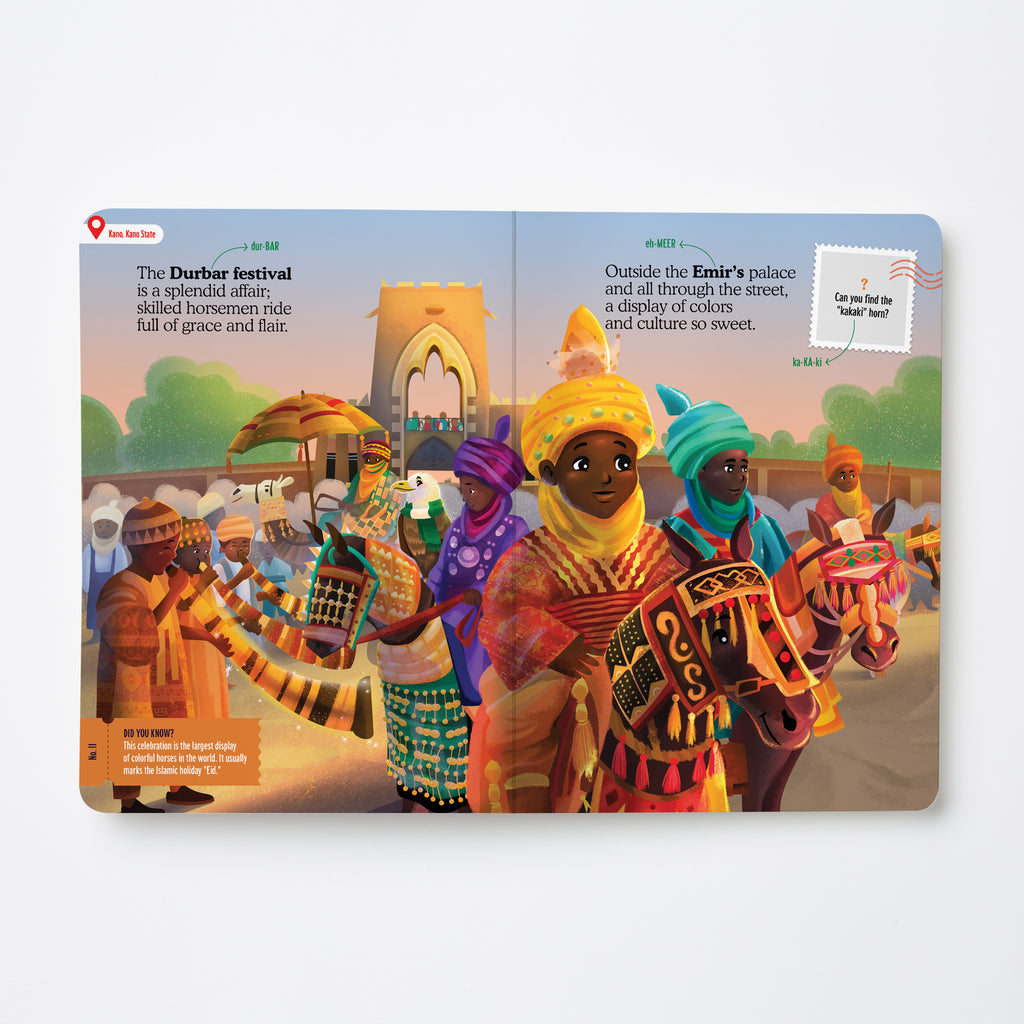The scene depicted in the image is a vibrant, outdoor, computer-generated animation taking place during the day. Centrally featured is an intricate portrayal of the Darbar Festival, a cultural celebration marked by a colorful parade. The main focus is on a group of horsemen, apparently of Middle Eastern or African descent, adorned in elaborate traditional attire. This includes black individuals riding horses decorated with ornate, multicolored coverings, particularly in shades of red, orange, and white. 

In the center foreground, a prominent figure sports a striking yellow turban and a matching red and yellow robe while mounted on a similarly adorned horse. To the right stands another person draped in a turquoise turban and robe, and to the left, one more individual with a purple turban and robe. Behind this central group, a festive atmosphere is conveyed with additional participants: a character holding a yellow and red umbrella, children in stocking caps blowing horns to herald the procession, and a person in orange mounted on a horse.

The background reveals a building with an arch and some trees, adding depth to the scene. The text accompanying the image reads, "The Darbar Festival is a splendid affair, skilled horsemen ride full of grace and flair," and, "Outside the Emir's palace and off of the street, a display of colors and culture so sweet." Additionally, there are playful elements like a stamp that challenges viewers to find a "khaki ham" and text in the top left corner noting the largest display of colorful horses in the world, usually marking the Islamic holiday, Eid. The image exudes a sense of celebration, diversity, and cultural richness, highlighting the festival's grandeur and festive ambiance.